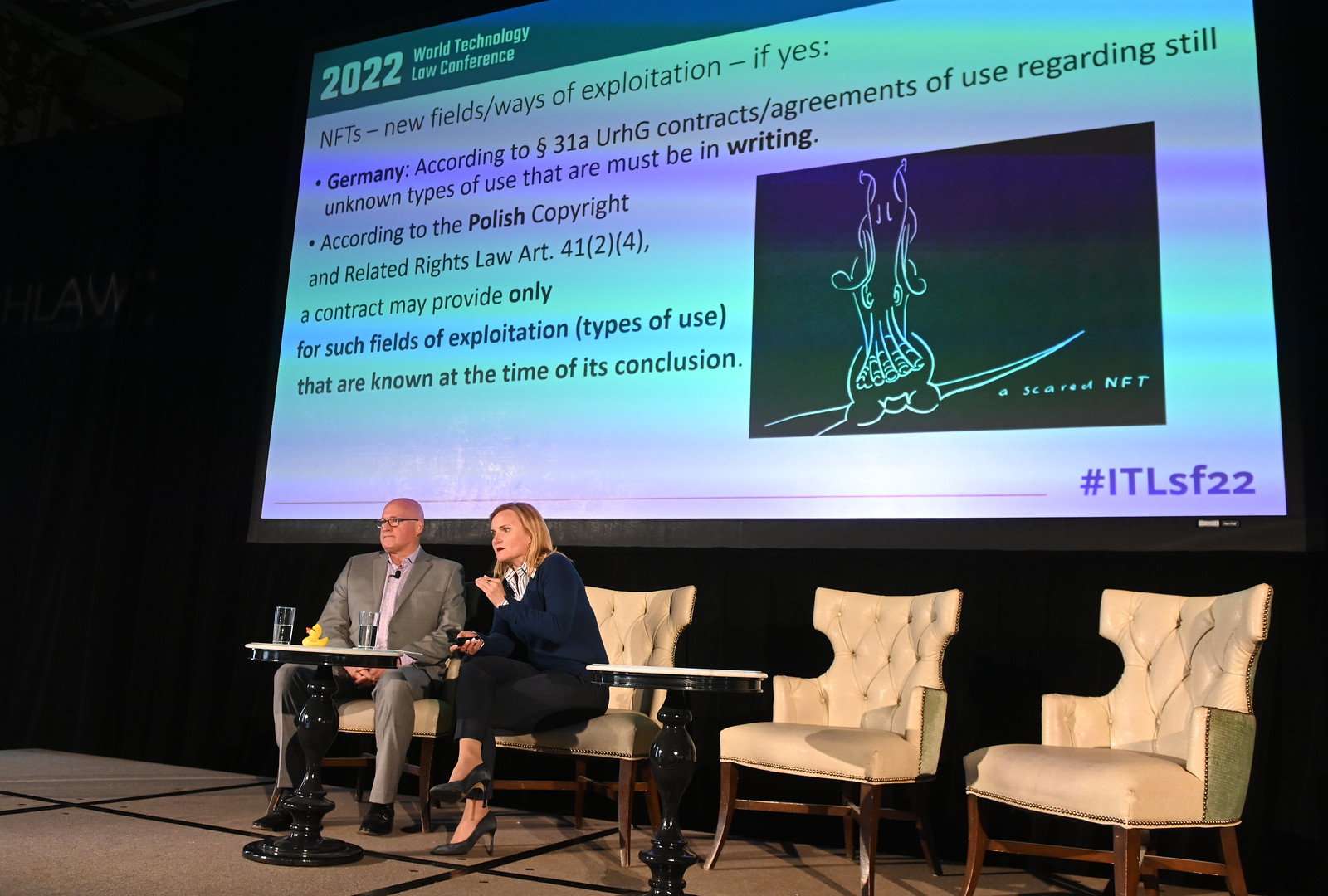The image depicts a stage setup at the 2022 World Technology Law Conference. On the stage, there are four cream-colored leather chairs with wooden legs, two of which are occupied. The two people seated are a bald, middle-aged man wearing an olive green or gray jacket over a light-colored shirt and pants, and a woman in a blue suit coat with black trousers, a white shirt, and black heels. The woman, possibly speaking, holds the projector remote. 

In front of them are tables with water glasses and a small yellow rubber duck. Behind them, a large screen displays a detailed slide about NFTs and their legal implications. The screen includes the conference title "2022 World Technology Law Conference" and sections like "NFTs: New Fields/Ways of Exploitation" and "Germany, according to 31A UrhG, contracts/agreements of use regarding still unknown types of use must be in writing." It also references the Polish Copyright and Related Rights Law, Article 41, with sections describing contractual provisions for fields of exploitation known at the time of conclusion. An image of a cat marked as a "scared NFT" and the hashtag #ITLSF22 are also visible on the screen.